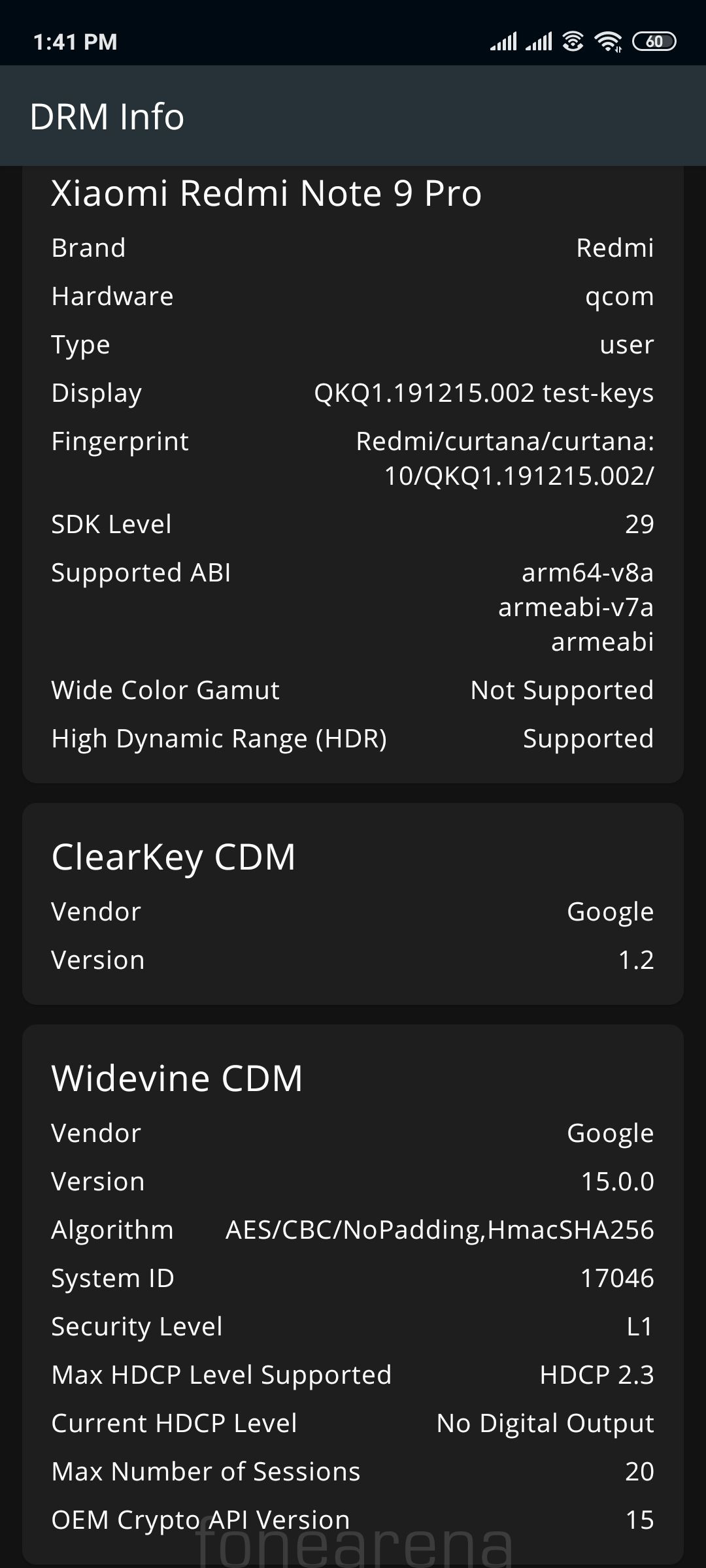The image is a screenshot of the DRM Info screen from a Xiaomi Redmi Note 9 Pro device, presenting detailed device specifications and DRM capabilities. The screen displays the following information:

- **Display**: QKQ1.191215.002 test-keys fingerprint
- **Software**: MIUI 12 based on Android 10
- **Supported ABI**: ARM64-V8A, ARMEMABI-V7A, ARMEABI
- **Wide Color Gamut**: Not Supported
- **High Dynamic Range (HDR)**: Supported
- **Clear Key CDM**: 
  - Vendor: Google
  - Version: 1.2
- **Widevine CDM**: 
  - Vendor: Google
  - Version: 15.0.0
  - Algorithm: AES/CBC/NoPadding
  - HMAC SHA-256
  - System ID: 17046
  - Security Level: L1
  - Max HDCP Level Supported: HDCP 2.3
  - Current HTTP Level: Not provided
  - Max Number of Sessions: 20
- **OEM Crypto API Versions**: Presented but details not provided

Additional screen details:
- The **battery icon** is at 60% charge.
- **WiFi signal** and **notification icons** are present in the upper right corner.
- The **time display** shows 1:41 PM.
- The background is dark with white text following a dark theme.
- **Text is highlighted in bold** for emphasis.
- A watermark at the bottom, potentially reading "Phone Arena", attributes the screenshot to the owner or source.

The screenshot encapsulates various Android elements and UI features, providing a comprehensive overview of the device's DRM capabilities and system details.